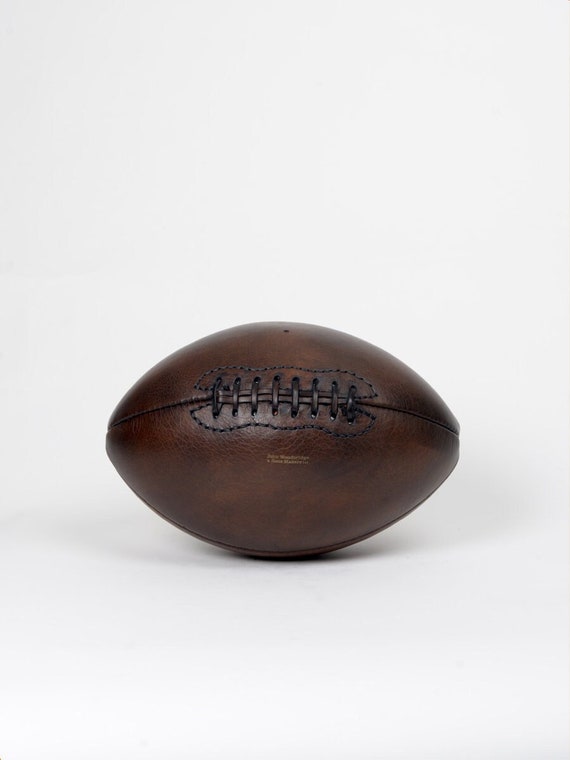This is a detailed photograph of a vintage American football, showcased against a plain white background. The football, made of leather, features a distinct almond or oval shape, which gives it a more old-fashioned appearance compared to modern versions. It has a dark brown color with a subtle red tint. Eight lines of stitching can be seen prominently down the center of the ball. Additionally, there are black markings flanking both sides of the seams, and below these seams, there is some yellow text, although it's too small and blurry to read clearly. A black circle is noticeable at the top of the football. The entire photograph is formatted vertically, with the football positioned slightly toward the bottom center. The plain white background and lack of additional text in the image focus all attention on the football itself.